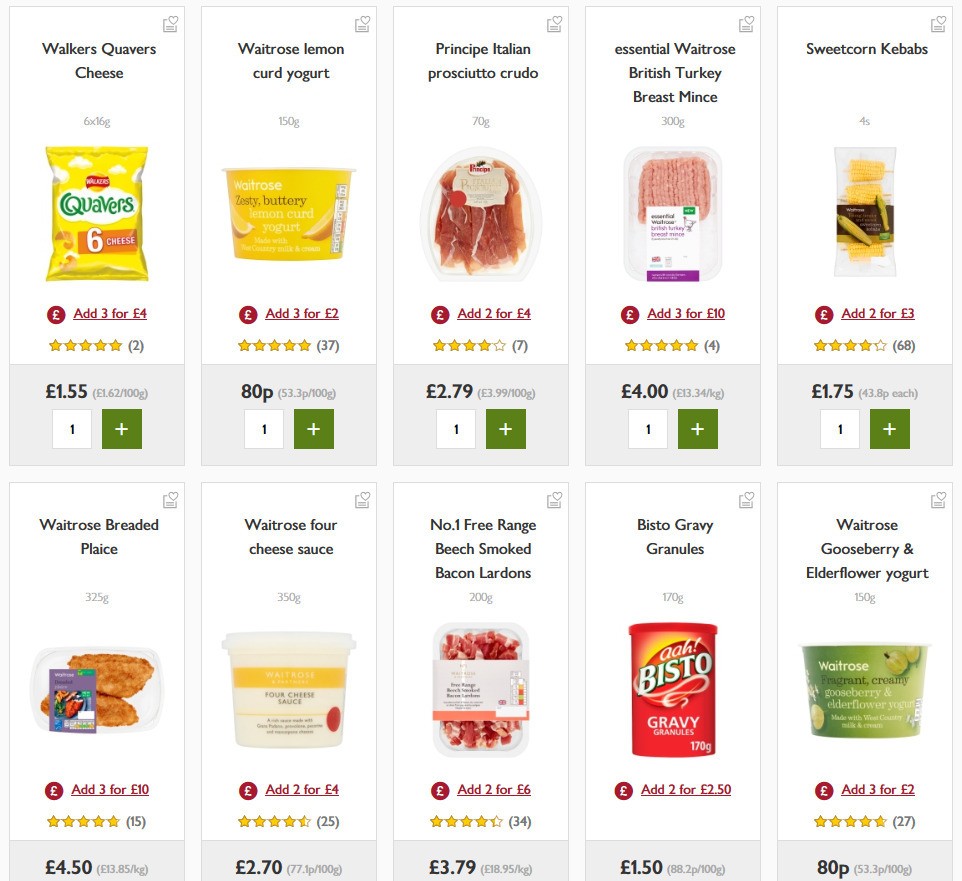The screenshot depicts a page from a UK-based grocery e-commerce site, showcasing various products. Each product listing includes multiple elements for ease of shopping:

1. **Product Information**: Each entry consists of the product name, accompanied by a high-quality image of the product.
2. **Weight and Pricing**: Details about the product’s weight are provided, along with pricing in pounds (£). 
3. **Special Offers and Add to Cart**: There’s a prominent “Add to Cart” button which allows customers to add items, including options like "Add 3 for £2". 
4. **Ratings and Reviews**: Beneath the product images, star ratings are displayed with the number of reviews in brackets.
5. **Main Price Highlight**: A lightly shaded box emphasizes the main price of each product.
6. **Quantity Control**: Customers can easily adjust quantities using a number input box, with a green button on the left featuring a white plus sign to increase the quantity.

The visible product listings are as follows:
- **Top Row**:
  1. Walker's Quaver's Cheese
  2. Waitrose Lemon Curd Yogurt
  3. Principe Italian Prosciutto Crudo
  4. Central Waitrose British Turkey Breast Minced
  5. Sweet Corn Kebabs

- **Bottom Row**:
  1. Waitrose Breaded Plaice
  2. Waitrose Four Cheese Sauce
  3. Number One Free-Range Beech Smoked Bacon Lardons
  4. Bisto Gravy Granules
  5. Waitrose Gooseberry and Elderflower Yogurt

This selection highlights the diversity of products available at the store, ranging from dairy and meats to condiments and snacks.